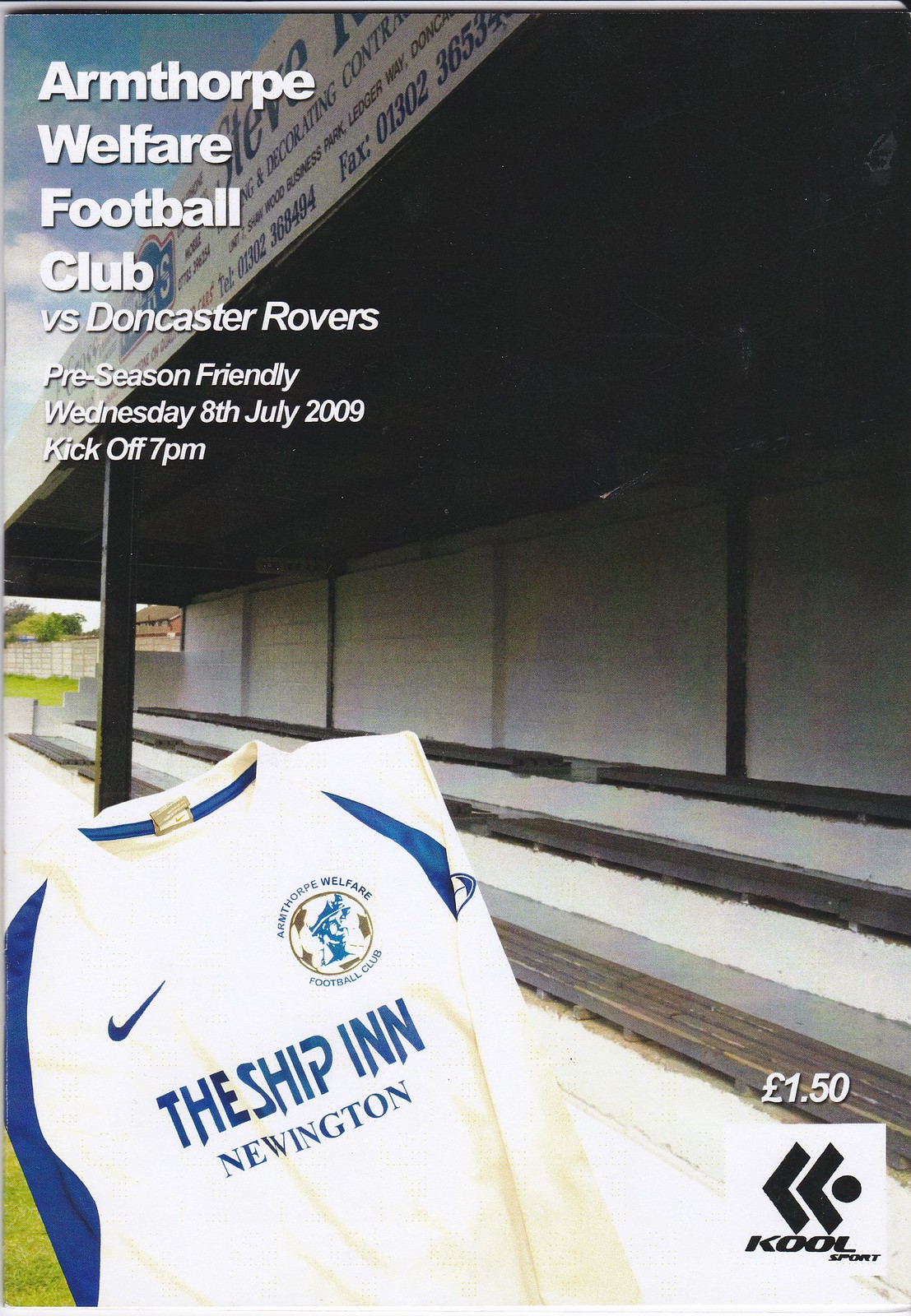The image appears to be the cover of a soccer program for a preseason friendly match between Armthorpe Welfare Football Club and Doncaster Rovers, scheduled for Wednesday, 8th July 2009, with a kickoff at 7 p.m. The main background of the cover depicts a dugout, featuring benches under an awning where players can sit. This area is detailed with elements resembling a train station platform, including dark-colored poles, a white wall, and a roof. Some grass and a blue sky are visible in the background.

Prominently displayed in the lower portion of the cover is an image of a white jersey with blue trim, bearing the text "The Ship Inn, Newington" in blue. The Armthorpe Welfare Football Club logo is also visible, depicting a soccer ball with an illustration of a miner's helmet equipped with a light. Nike's logo is featured on the jersey as well, emphasizing the sponsorship details.

In the lower right-hand corner, the program’s cost is listed as £1.50, adjacent to a sponsor's logo - Cool Sport, which includes black chevrons pointing left within a white box. The comprehensive details and combination of visual elements make it clear that this cover is not only informative but also captures the essence of the upcoming friendly match.